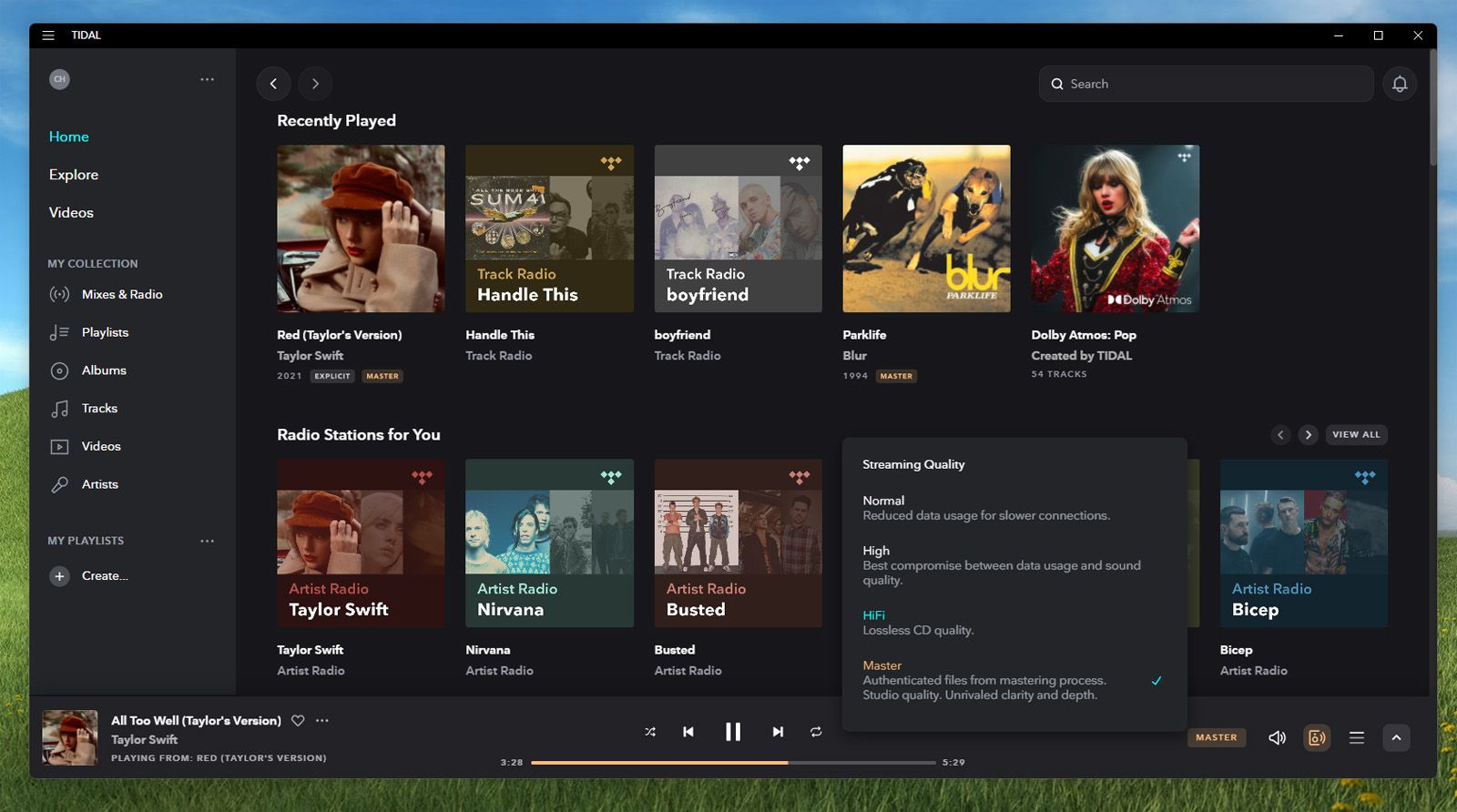The image showcases the Tidal music streaming platform, which bears resemblance to Spotify but features an orange color theme instead of green. At the top left corner, the Tidal logo is prominently displayed. The interface exhibits a modern layout with a black background accented by blue and orange hues. Visible on the screen are several album covers and trailers, including "Red (Taylor's Version)" by Taylor Swift and the playlist "Parklife" by Blur. The currently playing track is "All Too Well" by Taylor Swift. Additionally, there is a section for adjusting the streaming quality, offering options such as Normal, High, Hi-Fi, and Master, with the Master setting selected, indicating the highest audio quality available. The platform also includes various playlists and radio stations, enhancing the user’s music discovery experience.